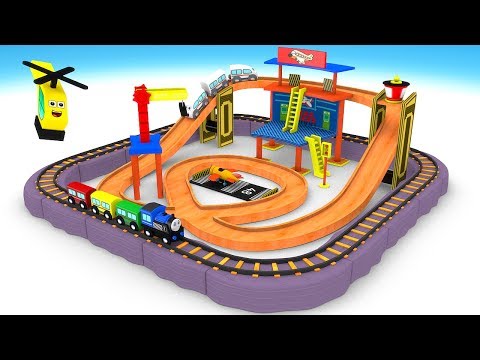In the image, we see a vibrant children's toy setup featuring a train and a car track arranged on a white background. The central focus is a blue engine, popularly known as Thomas the Train, complete with a friendly face. Thomas is followed by a sequence of colorful cars: green, yellow, and red. The train track itself is a square loop, bordered by black and yellow stripes, and made of thick purple block-like bricks.

Within this squared train track is an intricately designed orange race car track that ascends and descends a smooth hill, giving the appearance of a Hot Wheels track. The track, possibly mimicking an airport transport system, includes multiple levels connected by yellow ladders.

In the upper left corner of the image hovers a yellow toy helicopter, marked by a friendly face and black propellers. Additionally, there is a small takeoff track for an orange airplane, ready for a pretend flight. The combination of colors and elements creates a lively and dynamic scene, perfect for imaginative play.